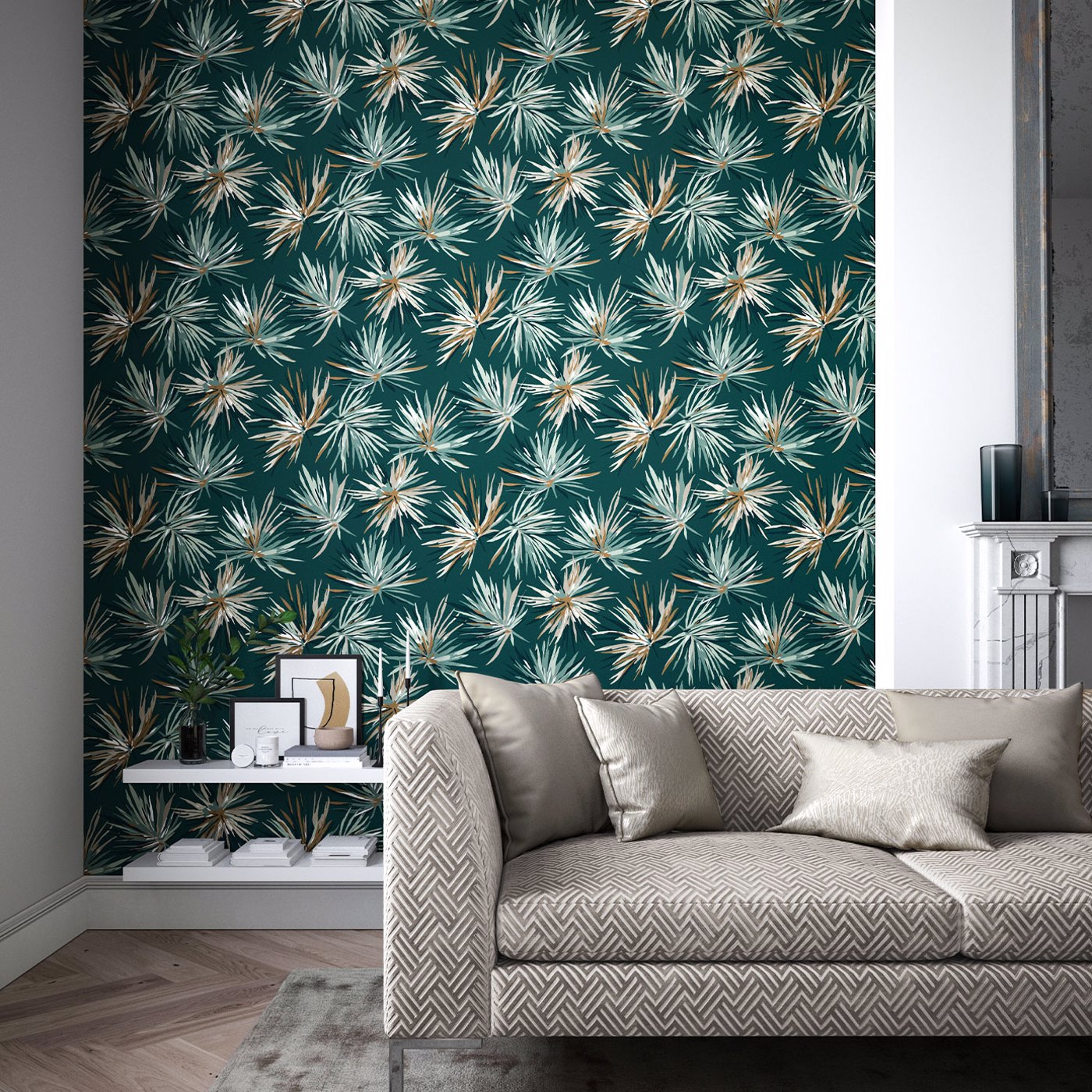The photograph features a meticulously organized and elegantly decorated living room, which exudes a luxurious and expensive ambiance, resembling a space often showcased in magazines or realtor advertisements. The focal point is a sophisticated beige or greyish-brown couch adorned with light brown, metallic-hued pillows, creating a cozy yet upscale atmosphere. Positioned beneath the couch, a stylish rug complements the wooden flooring. The backdrop includes a striking sage green and white wall, adorned with a pine-needle or floral-like wallpaper, embellished with delicate white and yellow accents. An array of white floating shelves lines the wall, displaying an assortment of decorative items, including candles, small statues, and framed pictures. Dominating the right-hand corner of the room is a pristine white fireplace, adding to the room's warmth and elegance. The overall aesthetic is one of immaculate cleanliness and artistic presentation, highlighting both comfort and refined taste.